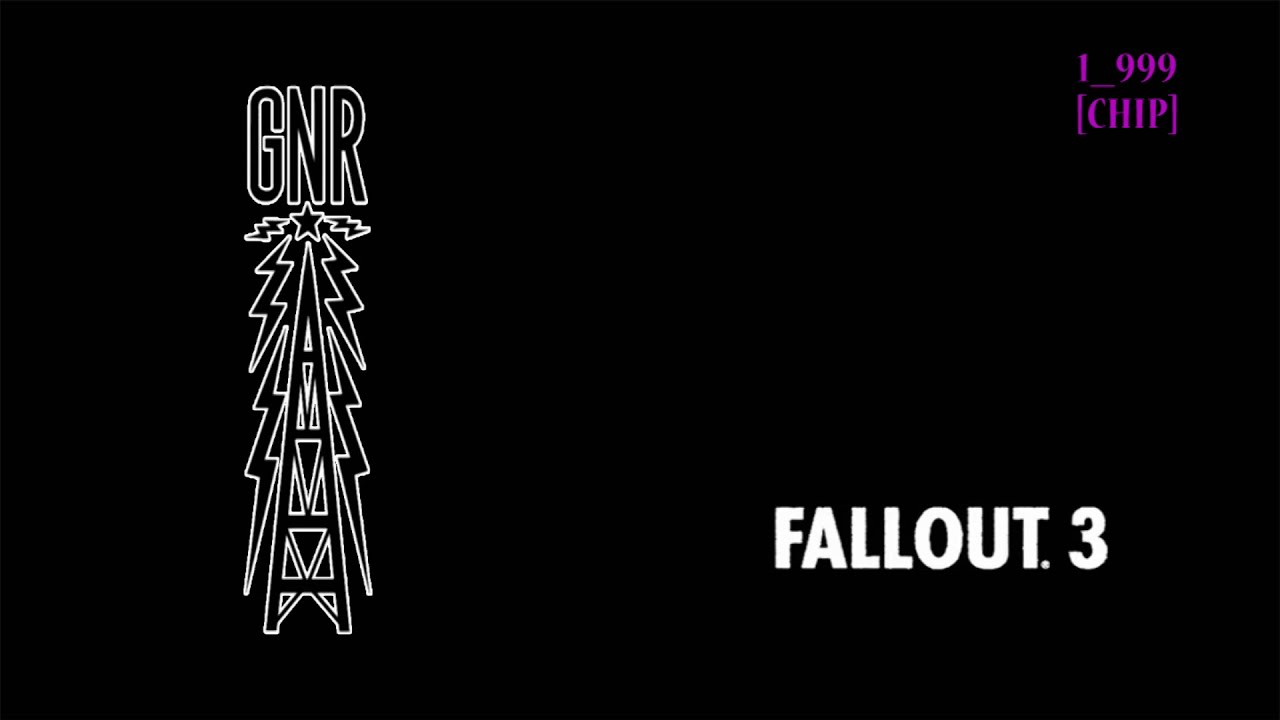The image features a stark black background, with several distinct elements arranged across it. In the upper right corner, in a purplish-pink font, it reads "1_999," and directly below that, enclosed in brackets, is "CHIP" in all caps. Both elements are positioned near the top-right edge. Dominating the bottom right corner is the text "FALLOUT.3" in large, bold white capital letters. On the left side, running vertically from top to bottom, is an intricate design: it starts with the capital letters "GNR" in black, outlined in white. Beneath this text is an image resembling a high-voltage power line or totem pole, with a star at the top and beams of lightning radiating downward. These elements, including the tower, star, and lightning bolts, are also rendered in black with white outlines. The overall layout gives the impression of a computer-generated promotional graphic or advertisement, primarily utilizing a monochromatic color scheme accented with purplish-pink text.